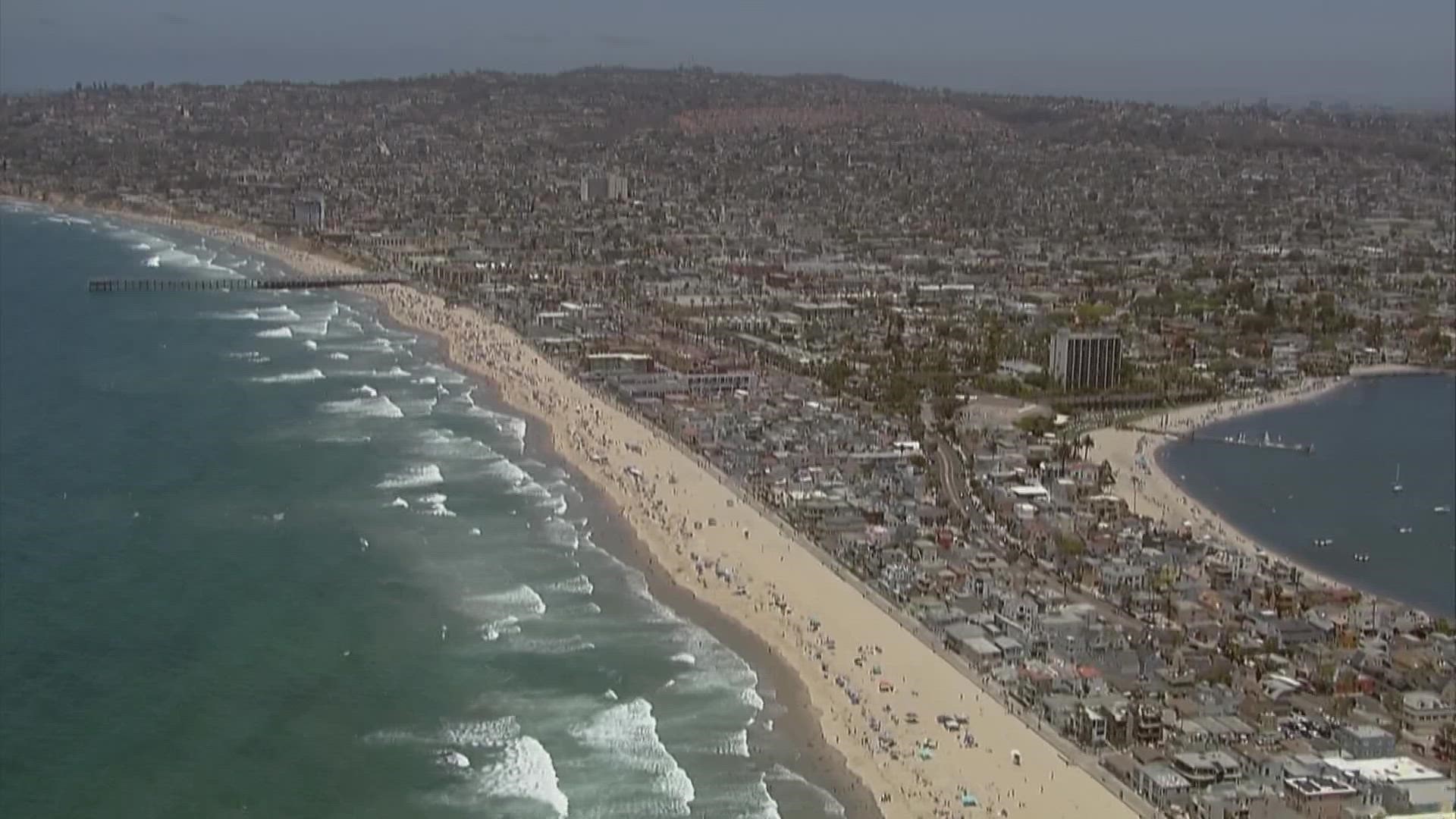An aerial photograph captures a picturesque city nestled on a beachfront, likely taken from a high vantage point such as a helicopter. The expansive ocean dominates the left side, its waves, adorned with white caps, gently crashing onto the extensive stretch of white sandy beach where numerous tiny figures, resembling ants, dot the shoreline. The beach extends along the bottom of the image, curving gently to the right. The left side of the photograph features a prominent pier jutting out into the ocean, with more water visible in the background and on the right side, creating the impression of an inlet or peninsula. 

This peninsula-like formation, possibly an island, showcases a mix of densely packed homes and buildings, with a few taller office structures hinting at a bustling yet vacation-like atmosphere. A second pier is visible extending into the water on the right side, where several small boats are seen floating. The picturesque scene is set against a slightly hazy sky, encapsulating the tranquility and vibrancy of this coastal city.